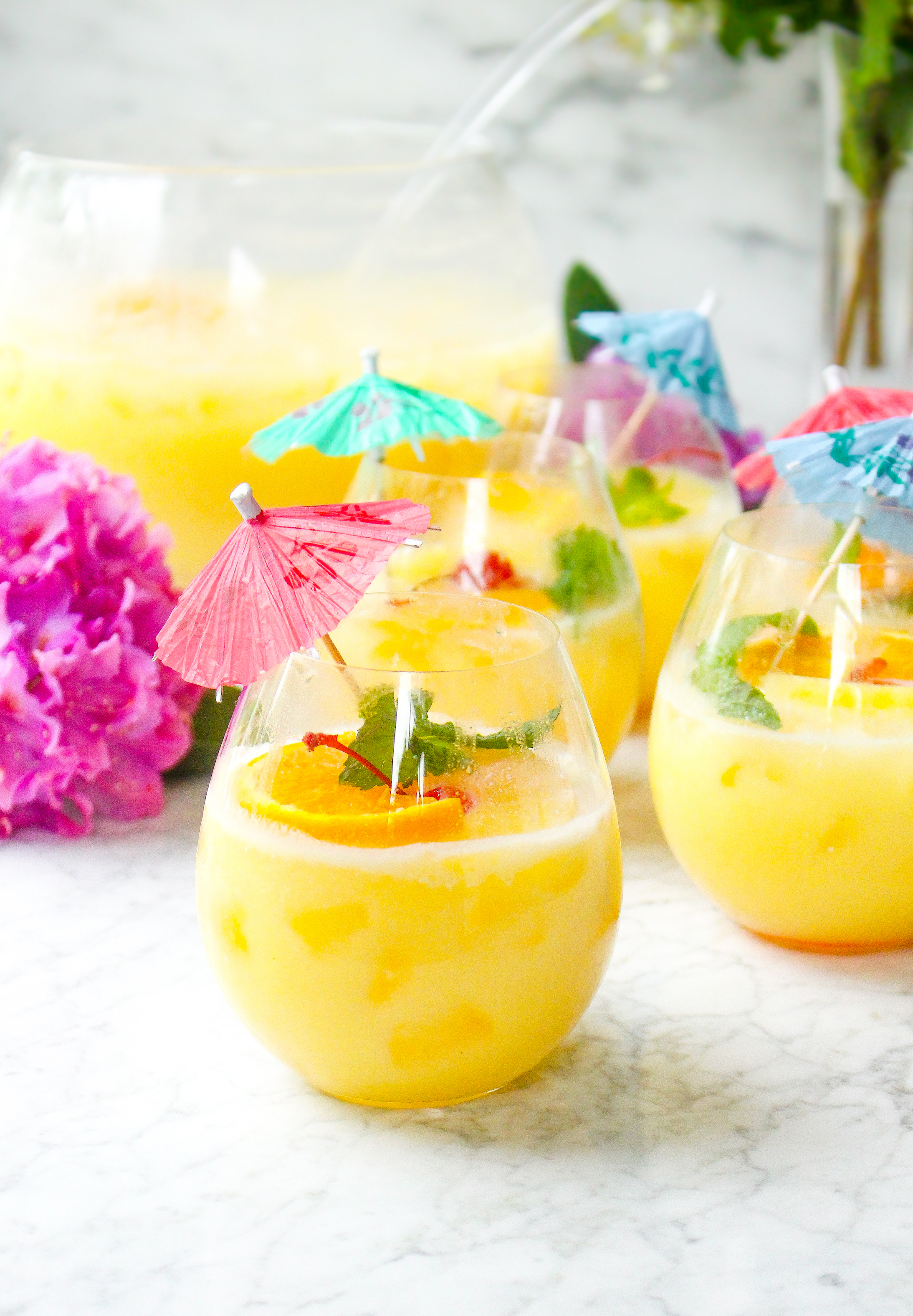The image features a full-color, vertically rectangular staged photograph of a tropical drink setup. The drinks are in flat-bottomed, clear glasses, not very tall, filled with a yellowish-orange liquid. Each glass contains ice cubes, a slice of orange, a maraschino cherry, and a mint sprig, topped with a colorful paper umbrella in shades of red, blue, pink, and green. The glasses are arranged on a marble surface, with a beautiful fuchsia flower and green leaves present to the left. In the upper right-hand corner, a green stem and leaves can be seen, though slightly out of focus. In the background, a bit blurry but still discernible, is a large punch bowl with a ladle, containing a similar yellowish concoction, enhancing the festive setting.